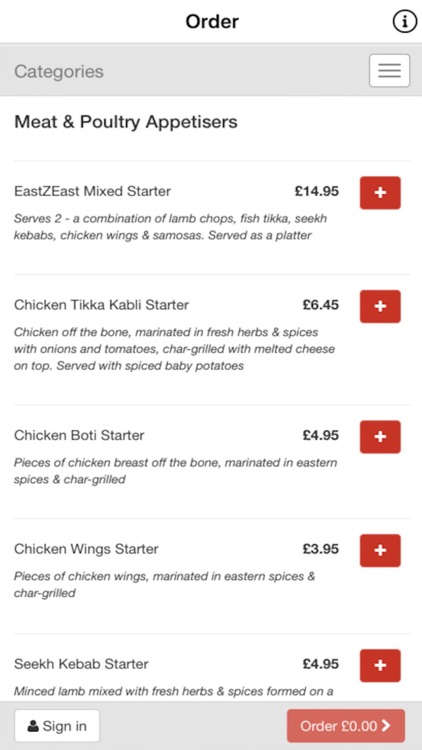A screenshot of an online menu from a British website is displayed. At the top of the page, the word "Order" is prominently featured. Below this heading is a list of meat and poultry appetizers, indicating British English spelling by using "appetisers" and listing prices in British pounds.

The menu highlights various starters, including the "East Z East Mixed Starter," which is a combination of lamb chops, fish tikka, and other items, priced at £15. Another item is the "Chicken Tikka Kabli Starter," costing £6.45. The menu also offers a "Chicken Wings Starter," which falls in a lower price range, along with a kebab item.

The background of the menu is white with black text, ensuring readability. A red "Order" button is located at the bottom right corner, currently indicating that no items have been added to the cart. A "Sign In" button is on the bottom left, and a "Menu" button is positioned at the top right. Each menu item has a red plus button next to it, allowing users to easily add items or specify quantities.